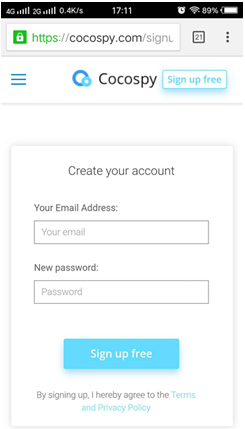This is a detailed screenshot of the signup page for CocoaSpy.com as viewed on a smartphone. At the top of the screen, indicators show a 4G connection, Wi-Fi status, a battery level of 89%, and a timestamp of 17:11. Icons for an alarm and signal strength are also present. Below this, the address bar is visible, along with a square icon containing the number 21 and a set of three horizontal dots. Further down, a hamburger menu icon is situated near the CocoaSpy logo, which consists of two connected circles—one larger and blue, the other smaller and baby blue.

Centered on the page, bold text encourages users to "Sign Up Free," followed by fields prompting for an email address and the creation of a new password. A button labeled "Sign Up Free" is prominently displayed. Text beneath this button indicates that by signing up, users agree to CocoaSpy's terms and privacy policy. This intricate layout and attention to detail typify the user-friendly design of CocoaSpy's registration interface.